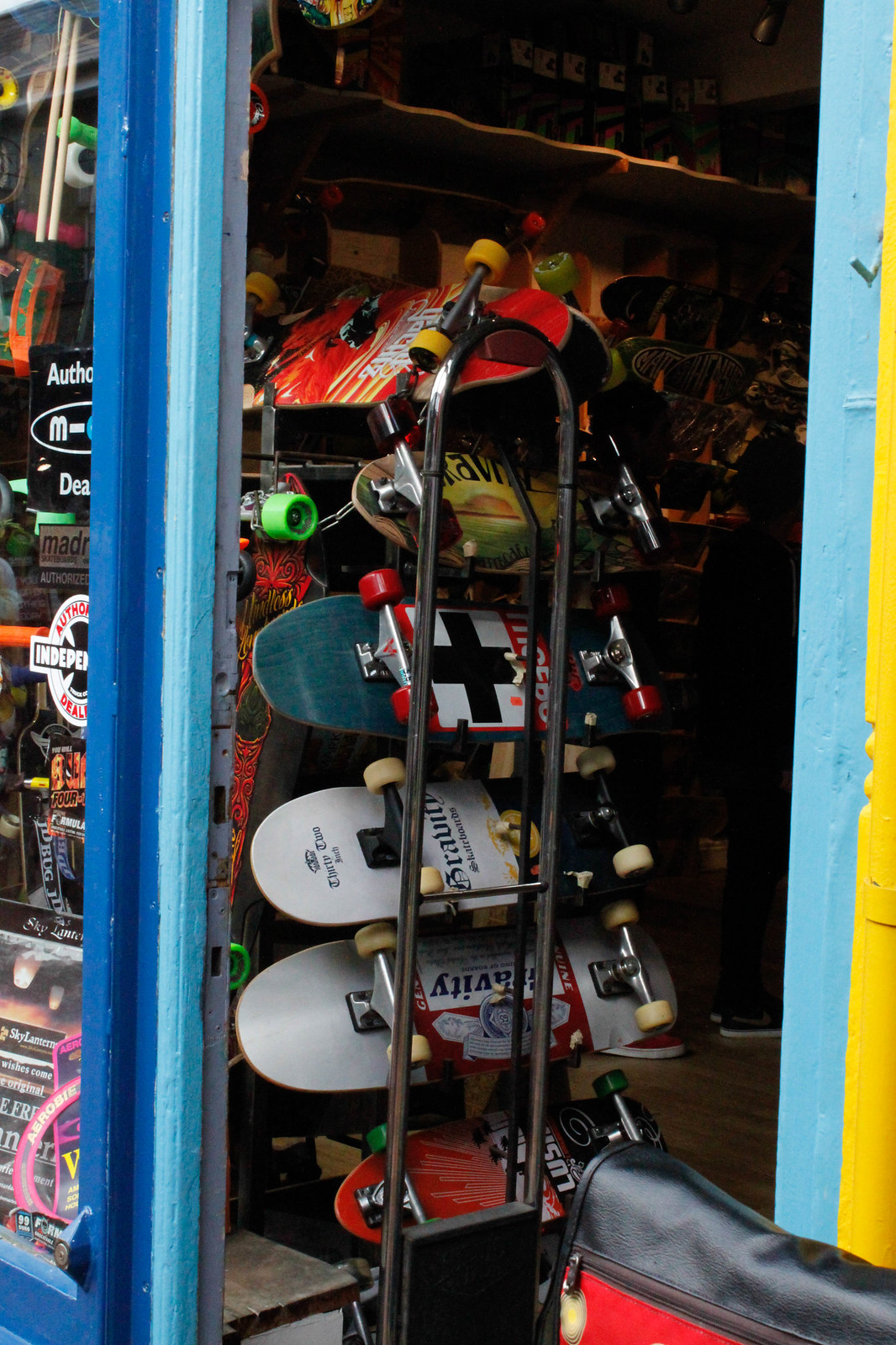The image is an outdoor color photograph capturing a window display of skateboards in a shop. Viewed from outside through the glass, the display features six skateboards arranged vertically on a chrome wire rack. The skateboards are stacked upside down at a slight 45-degree angle, with their wheels and trucks facing up. The skateboard designs exhibit various logos and colorful prints, though specific details are not entirely legible. Notably, the top skateboard is red with yellow wheels, followed by a green one with a scene and black wheels, a dark blue one with red wheels and a cross, a navy, white, and gold deck with "32" and an emblem, another resembling a Budweiser design but labeled differently, and a mostly red board with black and green wheels. The setting includes a light and dark blue corner post of the building on the far left, alongside a pane of the display window. The doorway to the right features light blue trim, giving a peek into the slightly dark interior where more skateboards and shop items are faintly visible.